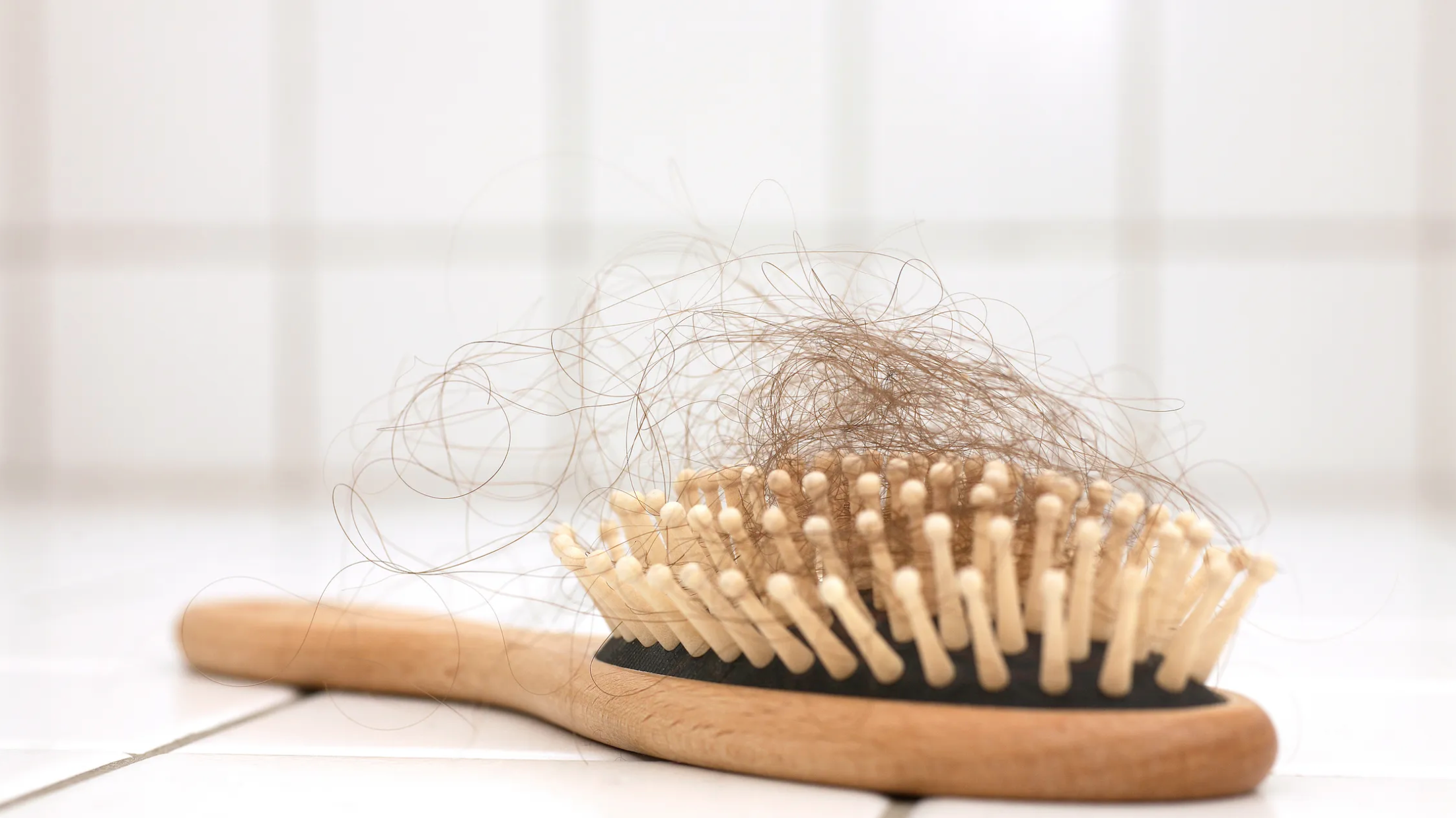A full-color photograph, clearly staged, captures a well-used wooden hairbrush laying on a white tile surface, with a white tile wall in the blurred background. The brush, positioned with its brown wooden handle at an angle towards the left and slightly back, features thick, beige plastic bristles with rounded tips emerging from a black base. Multiple rows of these bristles are visible, and tangled within them is a substantial amount of thin brown hair, clumped primarily in the center and extending out and over the handle. The white tiles have dark gray or black grout, creating a contrast that enhances the details of the brush and the hair entangled in it.